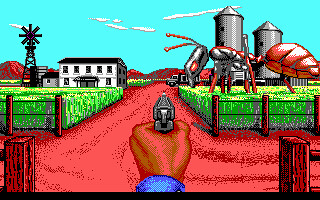This is a detailed visual from a computer game, characterized by its simplistic and flat graphics. The scene is set outdoors, dominated by a vivid red road that splits into two directions. On either side of this road, lush green grass is visible, bordered by a fence with a red post in front. To the left, a two-storey house with white walls stands at the edge of the grassy area, accompanied by a nearby pylon and a backdrop of a red mountain. To the right, the scene features two grey, round towers with pointed tops, resembling large monstrous insects with antennas oriented towards the road and a noticeable red humped back at the far right edge. The middle of the scene is occupied by a hand with darkish orange skin, holding a gun; the hand emerges from the edge of a blue top or shirt. Above, the sky is a clear blue, dotted with a few white clouds, adding to the serene yet surreal ambiance of the game environment.